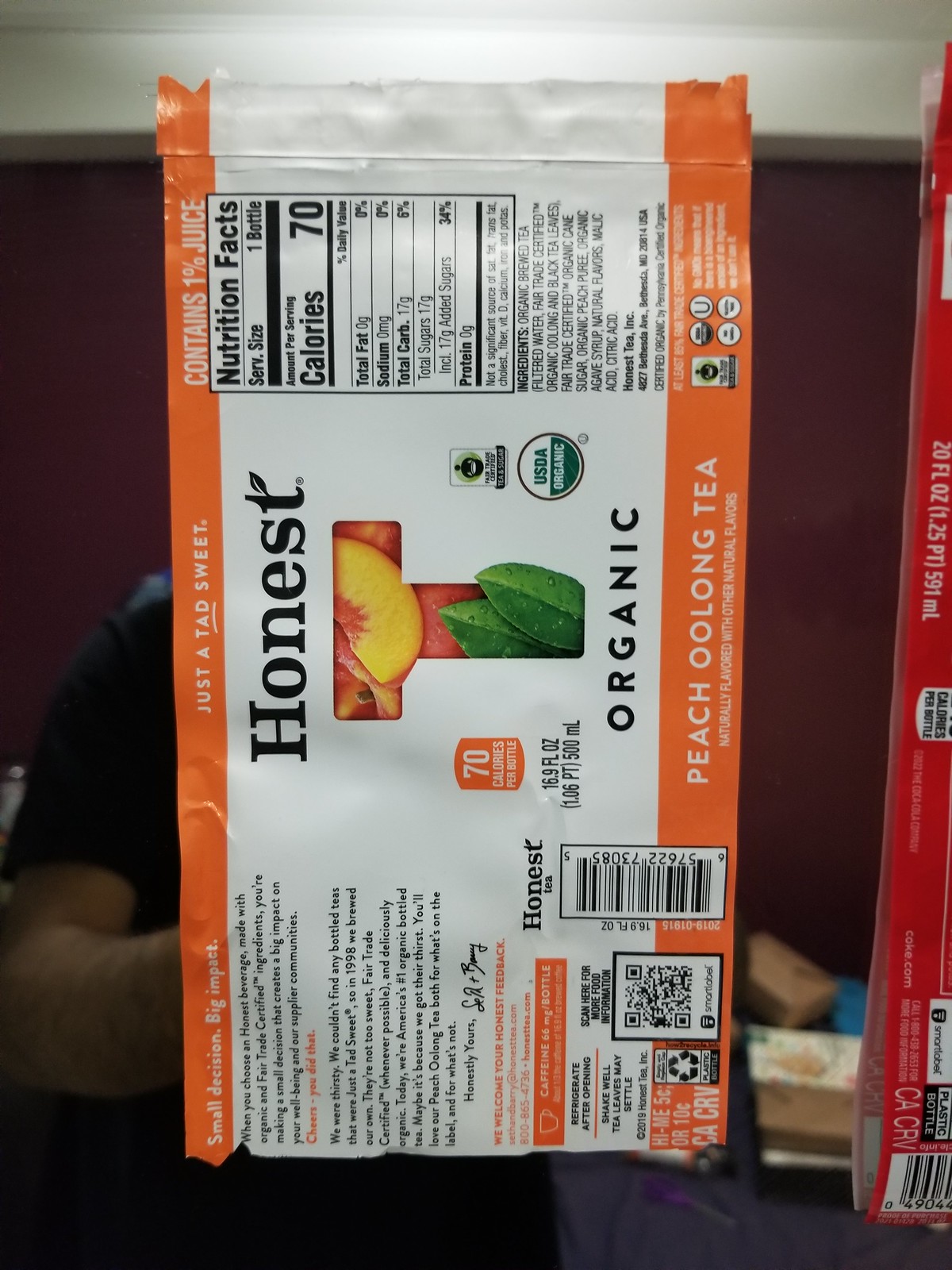This image features a horizontally-oriented label from an Honest Organic Peach Oolong Tea bottle, affixed to a mirror. The top of the label is to the left, and the bottom is to the right. The label dominates the left side of the image, stretching from the top to the bottom, and is primarily orange with white lettering, featuring a central white section. In the middle of this white section, there is a large T made up of fruits and vegetables, and beneath it, the words "organic" and "honest" in black lettering. 

Above the white section are the nutritional facts, which mention details like the 70 calories and no sodium content. Further to the right on the label, there's information about the product, including ingredients and a statement reading "Honestly Yours," likely attributed to the founder. The orange color of the label is highlighted at both the top and the bottom, signifying the peach flavor.

Near the right edge of the mirror, you can glimpse another red label hanging, mostly out of the frame. The mirror's reflection shows a red wall and packages that appear to be dark brown and light brown boxes, along with a blue cover on a bed. Additionally, there is a person's arm visible; they are wearing a black shirt, and their hand is partially obscured, positioned behind the label. The label also includes a barcode and the USDA organic symbol, confirming its organic certification.